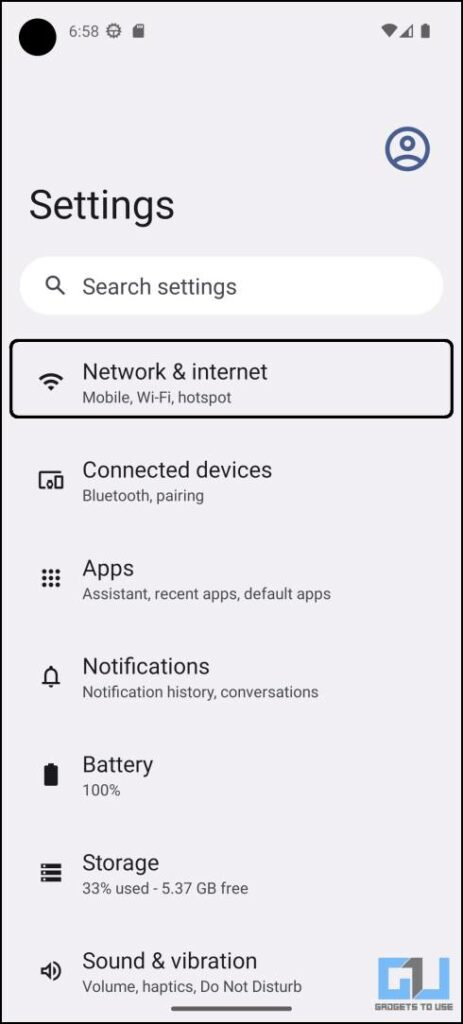This is a detailed caption for the given image:

---

Screenshot of a smartphone's settings page, timestamped at 6:58. The device shows strong Wi-Fi connectivity and a fully charged battery. The page title reads "Settings," and a search box for settings is available at the top. 

The sidebar contains several vertical tabs with associated icons. The currently selected tab is "Network & Internet," which includes options for Mobile and Wi-Fi hotspot settings. 

- **Connected Devices**: Features a device icon, includes Bluetooth pairing options.
- **Apps**: Identified by a grid of ellipses, covers Assistant, recent apps, and default apps settings.
- **Notifications**: Marked with a bell icon, includes notification history and conversations.
- **Battery**: Represented by a battery icon, shows the battery is at 100%.
- **Storage**: Displayed with a three-bar icon, indicates 33% used, 5.37 GB free.
- **Sound & Vibration**: Indicated by a speaker or earbud icon, includes settings for volume, haptics, and Do Not Disturb mode.

The bottom of the page appears to reference a site or application with the initials "GU," but the full name is not readable.

---

This caption provides a comprehensive description of each element shown in the screenshot.